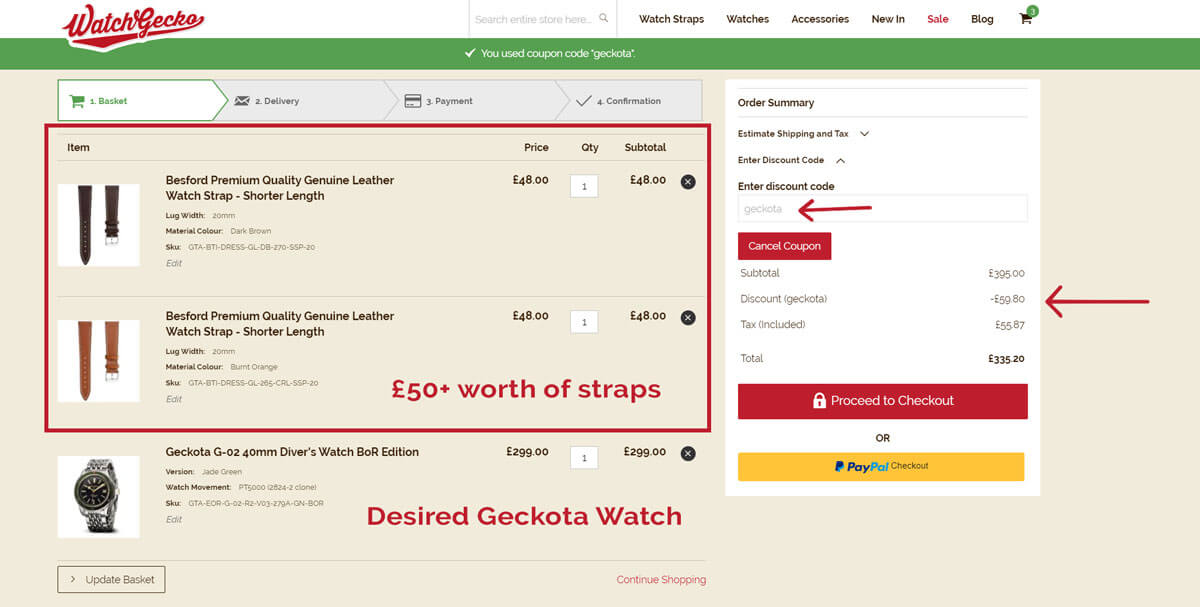This is a detailed screenshot of a web page from Watch Gecko. At the top of the page, there is a white navigation bar featuring the green logo "Watch Gecko" accompanied by a green stripe underneath. To the right of the logo, there is a search field with the placeholder text "Search entire store here" in gray font, alongside a gray magnifying glass icon. Further to the right, there are clickable menu options labeled: "Watch Straps," "Watches," "Accessories," "New," "Sale," and "Blog." At the far right end of the navigation bar, there is a black shopping cart icon with a badge indicating that there are three items in the cart.

The main content of the page below the navigation bar has a light green background. The current view shows the contents of the user's shopping cart, which contains: 

1. A Bedford Premium Quality Genuine Leather Watch Strap (Shorter Length) in black, priced at $48.
2. Another Bedford Premium Quality Genuine Leather Watch Strap (Shorter Length) in brown, also priced at $48.
3. Additional straps worth $50.
4. A watch listed as "Desired GECKO TELL Watch," priced at $300.